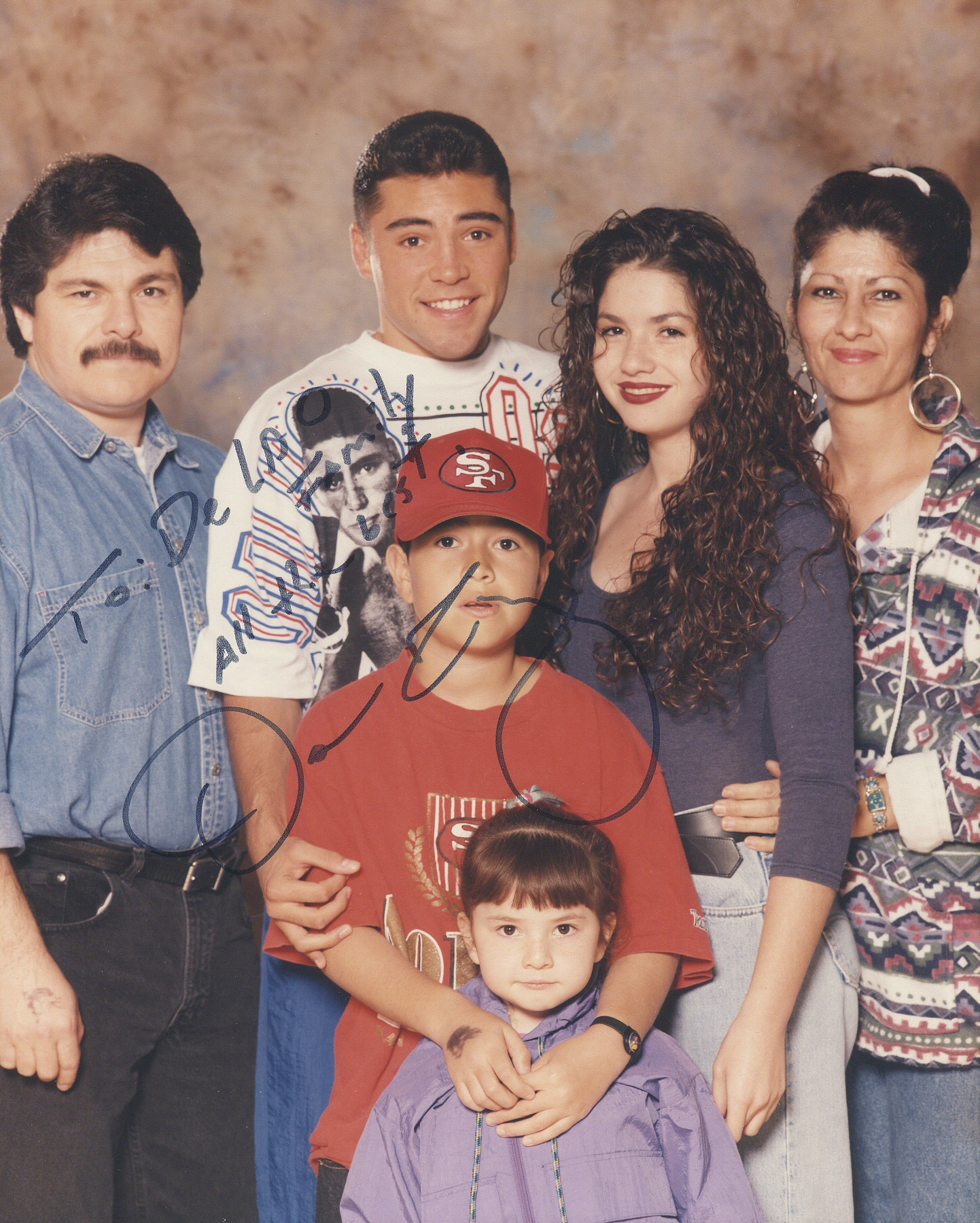This is a photograph of Oscar De La Hoya and his family, likely taken several years ago. The group consists of six people of varying ages, standing closely together and looking towards the camera. Oscar De La Hoya, recognizable with his short black hair and mustache, is second from the left. He is wearing a white shirt and jeans. On the extreme left stands an older man with dark hair and a mustache, clad in a blue shirt and dark pants, who has his arm around a woman. This woman, with long curly hair and wearing a colorful sweater, stands next to another younger woman who has a gray blouse and long curly hair flowing down her front. On the far right is another older woman dressed in a printed blouse and blue pants, her hair pulled back with a headband. In front of them are two children: a boy, almost a teenager, wearing a red San Francisco Giants cap and a matching red t-shirt, with his hands resting on the shoulders of a young girl in a purple shirt. The little girl, with bangs and dark brown hair, is looking straight ahead with a round face. The image appears to be autographed, indicating it might have been dedicated or given to someone.